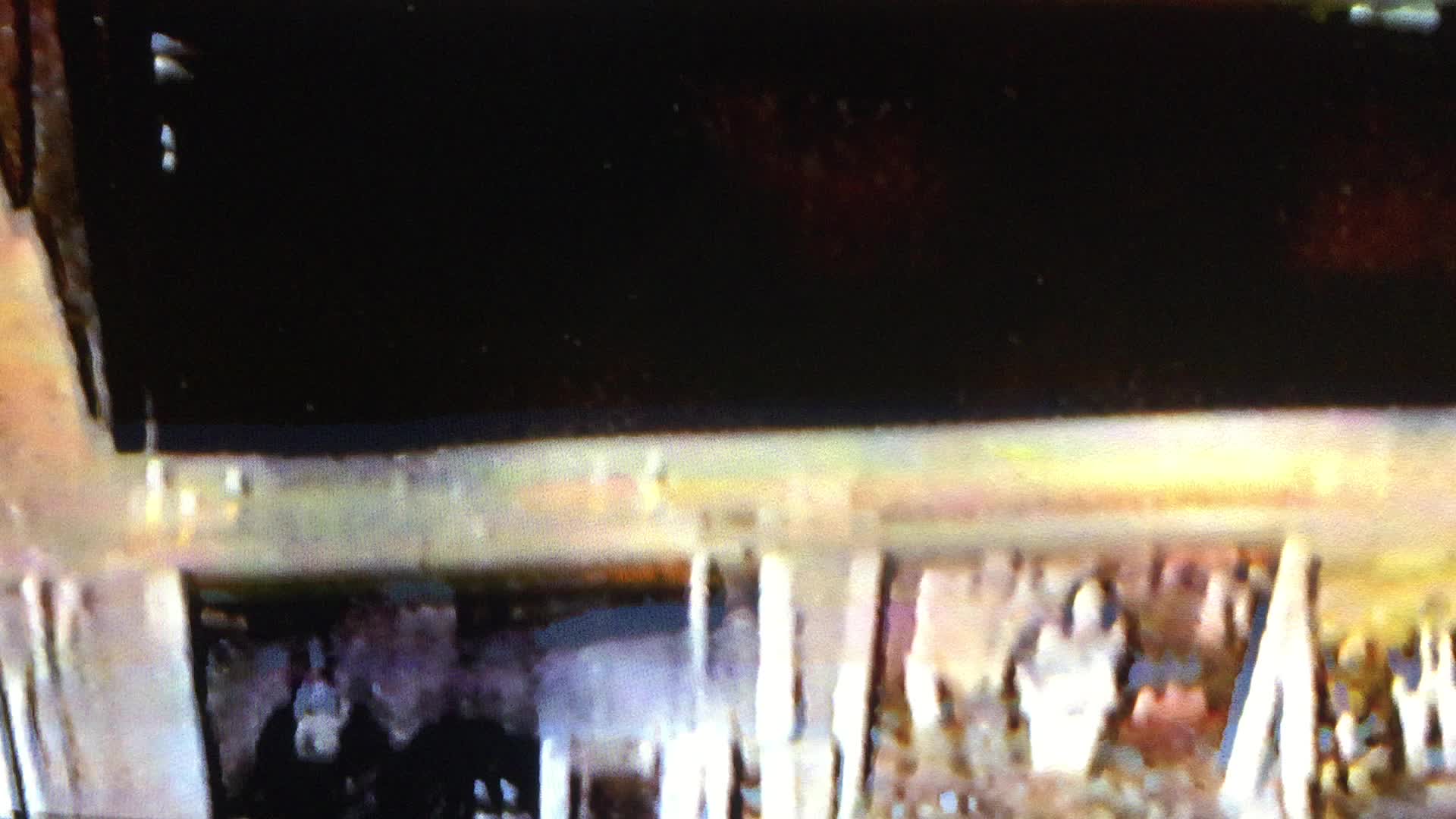This image is notably blurry, but several discernible shapes and colors offer some insight into its contents. The top section of the photograph is predominantly black, interspersed with occasional dark reddish-brown hues. Horizontally bisecting the image is a prominent stone beam, contributing to a sense of division within the scene. Additional stone elements are visible along the left-hand side, with what appears to be embedded objects or rust within the stone, adding texture and complexity.

The composition seems segmented into three distinct areas:
1. The bottom left section features a predominantly black background, accented with grayish rocks that subtly emerge.
2. The middle segment has a reddish backdrop, showing parts of white stone on the left and transitioning into gray at the bottom.
3. The bottom right section reveals a yellowish tone, with the presence of more white stone.

Despite the blur, the interplay of these colors and textures creates a segmented yet intriguingly varied visual narrative.